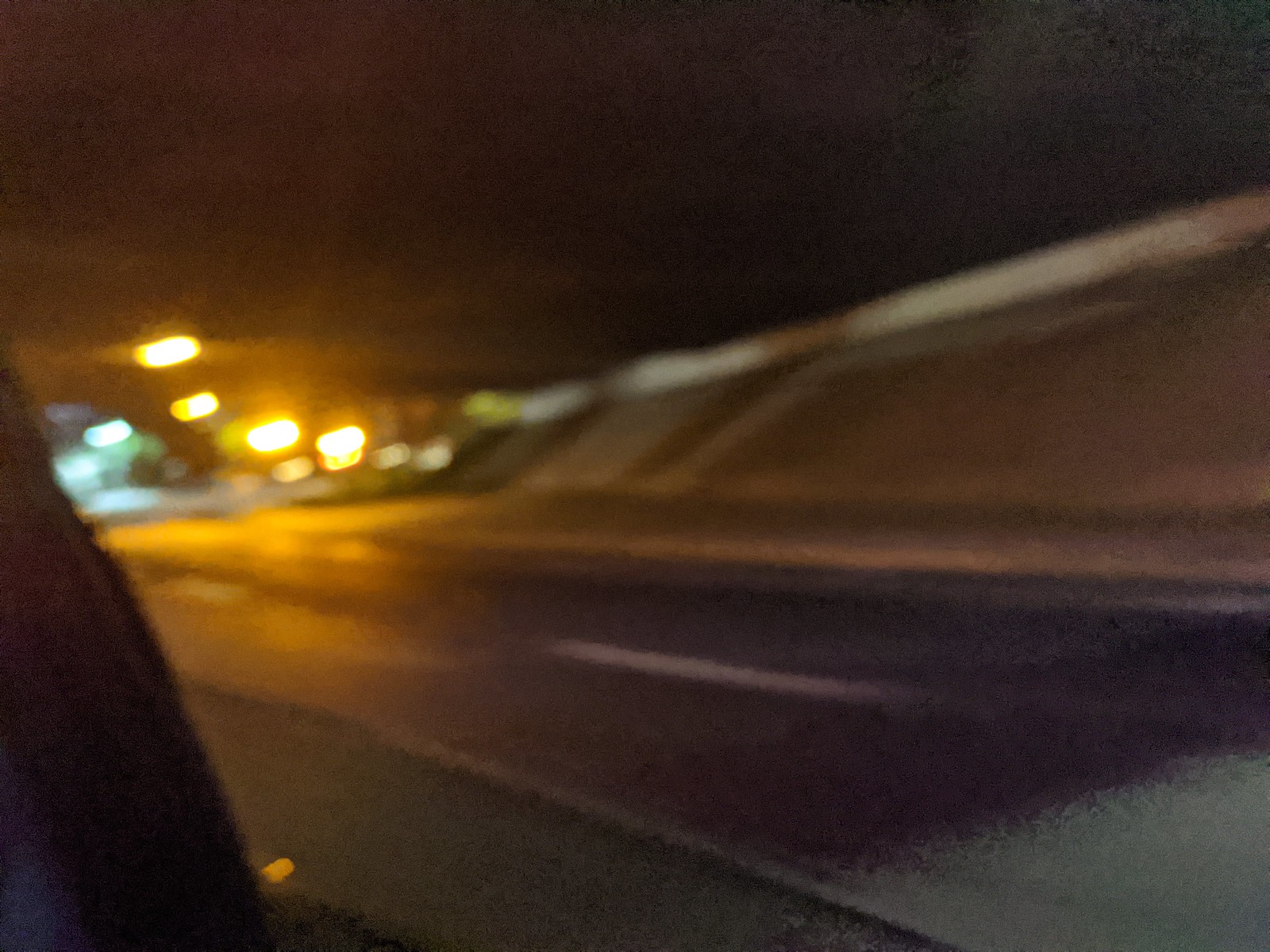A horizontally rectangular, extremely blurry photograph likely taken from within a moving vehicle captures a fleeting moment on a roadway. In the lower left corner, part of the vehicle's frame is partially visible, hinting at its presence. The image shows two lanes of a road, separated by a white lane marker. On the right side, a steep wall dominates the frame, while the top portion is engulfed in darkness, suggesting the vehicle is traveling under an overpass. Toward the left and down the road, a series of bright yellow lights, presumably streetlights, punctuate the scene, their glow softened by the motion blur.